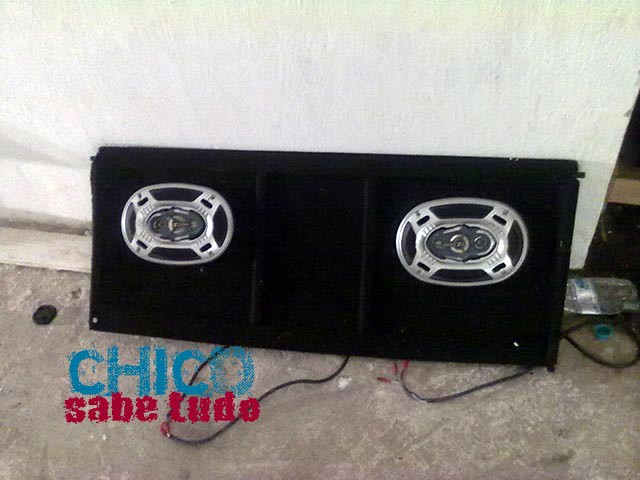In the image, a rectangular black boom box is positioned vertically against a light gray, nearly white, plaster wall. The boom box, featuring two side-mounted oval-shaped speakers with light gray centers and smaller circles or silver spokes within them, dominates the center of the scene. Two black cords emerge from its base, stretching across the gray cement floor. Blue text on the boom box reads "Chico," while reddish text below it reads "Sabe Ludo." To the right, a clear, flattened plastic beverage bottle with a light blue cap lies discarded on the ground, adding an element of debris to the otherwise stark setting.